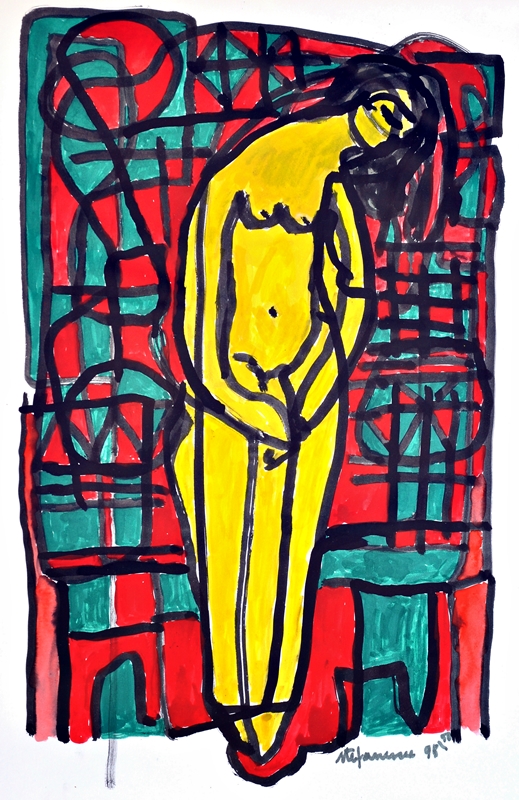This piece is an abstract modern illustration of a nude woman rendered primarily in yellow hues. The woman is depicted with long black hair that frames her bowed head, casting her gaze towards the right side of the composition as though she is looking downwards in a contemplative or shy manner. Her form is outlined in black, and her breasts, navel, and hands – which are folded demurely in front of her pelvis – are distinctly visible.

The background is a dynamic patchwork resembling a stained glass window, composed of irregular, geometric shapes in shades of red, green, blue, pink, and black. These shapes, outlined in black, add a vibrant yet chaotic energy to the scene. Black lines create a structured yet irregular pattern across the backdrop, enhancing its stained-glass aesthetic.

In the bottom right of the image, there is an illegible scribbled signature with the characters "m-i-f-a-n-a-n-u" and the notation "98," suggesting the year 1998. Additionally, there is an indication "98 out of 270" implying that this might be a limited edition print. The artist's identity remains unclear due to the indistinct signature.